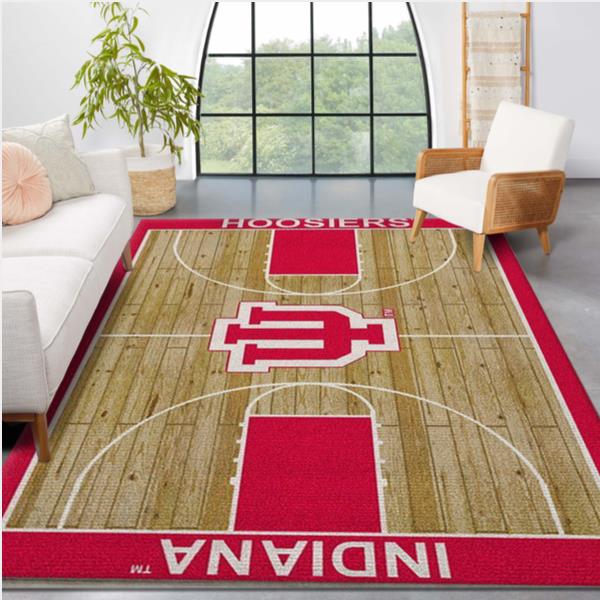This color photograph showcases an indoor living space, potentially a living room or sunroom, with a polished gray cement floor. The focal point is an area rug designed to resemble an Indiana Hoosiers basketball court, featuring a graphic hardwood court with a red border. At the top, "Hoosiers" is written in white, while "Indiana TM" appears at the bottom, and the center court displays the "IU" logo.

The left side of the room features a white two-seat sofa adorned with a gray square pillow and a pink round pillow. A green plant partially visible ahead of the sofa complements the space. On the right side, there's a small side chair with white cushions, rattan arms, and wooden feet. Adjacent to the sofa, a woven basket houses an olive tree.

Dominating the back wall is a grand arched window framed in black wrought iron, consisting of 12 glass panes, partially revealing a view of trees outside. To the right of this window is a blanket ladder against the wall, holding a cream-colored blanket. Additionally, a wooden, bookless bookcase adds a rustic touch to the room.